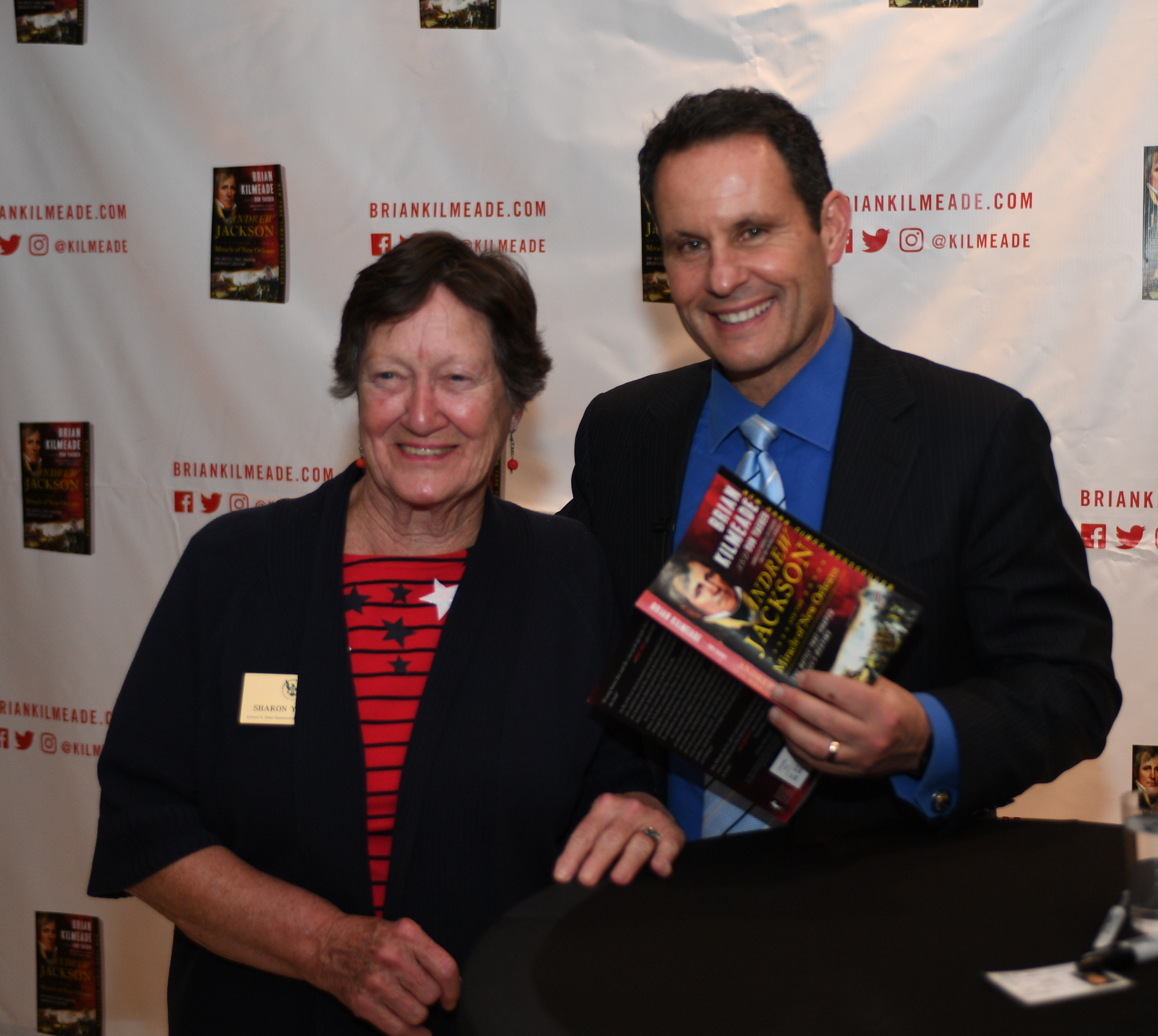At a book signing event, an author stands against a white curtain backdrop adorned with the repeating logo "briankillme.com" and images of a book. The man, dressed in a dark suit paired with a dark blue shirt and a silvery tie, smiles warmly at the camera. He has short dark hair and, with his left hand, is holding open a paperback book titled "Andrew Jackson," featuring his name on the cover, suggesting he is the author. A table to his right holds a pen, hinting at his recent or ongoing signing activities. Beside him, a woman stands close, clearly posing with him for an event photograph. She is dressed in a dark jacket over a distinctive red top with narrow black horizontal lines and scattered black stars at the top. The image captures the congenial atmosphere of the book signing event.